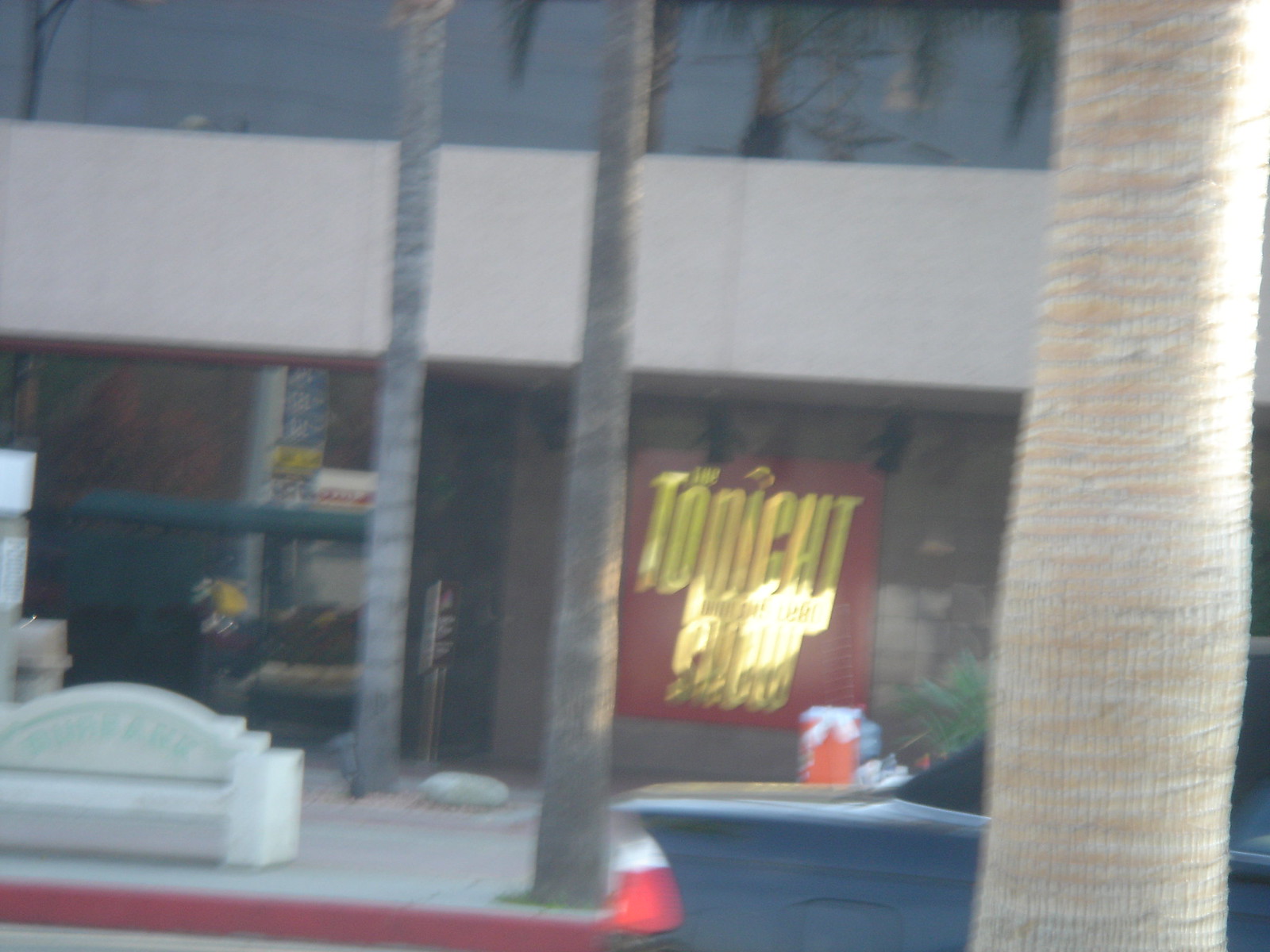The image portrays a blurry exterior view of a multi-level building, possibly a furniture store or an official establishment. The building façade features a reflective black window at the top, followed by a wide strip of light-colored concrete, and a dark brown section at the bottom. Dominating the right side of the building is a prominent red sign with yellow lettering that reads "Tonight," but the rest of the text is obscured by a reflection.

The foreground features a sidewalk with a white couch surprisingly placed on it near a tree trunk that is painted white. The curb at the front is painted red. In the middleground, a row of trees extends from right to left, with the main tree in the center showcasing a dark gray trunk, and another lighter gray trunk situated behind it to the left. Near the left edge of the photo, there is a white bench elevated on a white surface. Additionally, the corner of what appears to be a blue car or possibly a chair is visible near the white tree.

In the background, part of a street is visible with a car driving along it, described as either black or very dark in color. A trash can and a sign are also present on the sidewalk, alongside a concrete ledge and a brown wall further back. The overall scene is quite indistinct due to the blurriness of the image, making it difficult to capture more specific details.